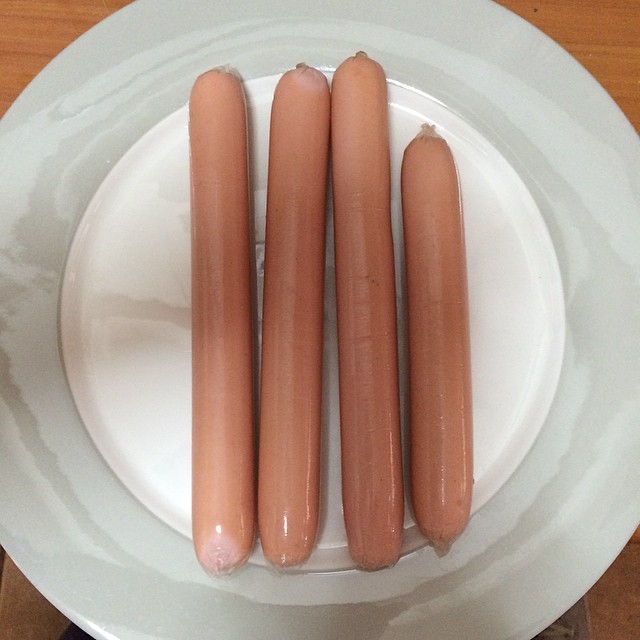The image features a simple, yet detailed scene of four uncooked hot dogs arranged vertically on a ceramic plate. The plate has a distinctive gray border with subtle white swirl patterns, and the interior is white. The hot dogs are a vibrant pink, indicative of their uncooked state, and they appear wet and shiny as though they have been recently rinsed or boiled. Three of the hot dogs on the left are nearly identical in length, while the one on the far right is slightly shorter and has a more pronounced casing. The plate rests on a medium to dark brown wooden surface, which can be seen peeking through the corners of the image, suggesting the plate is placed on a table. There are knots visible at the ends of the hot dogs, showing how they were packed. A partial, unreadable image or text lies beneath the hot dogs on the plate, adding a slight touch of intrigue to the otherwise straightforward composition.